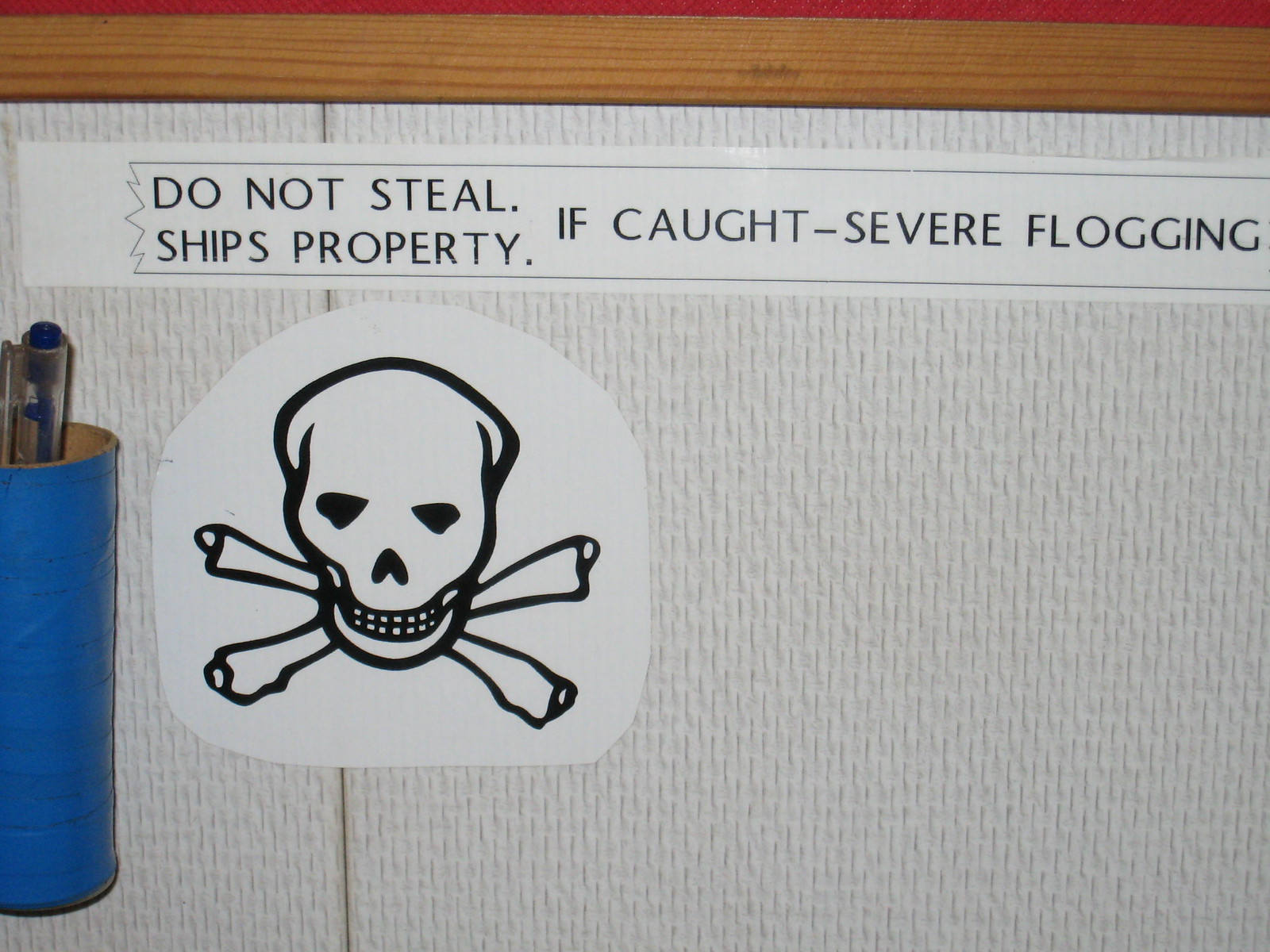The image shows a white mat or wall with a printed banner at the top that reads, "Do not steal ship's property if caught severe flogging" in black text. Below the banner, there is an amateurish drawing of a skull and crossbones, symbolizing danger or death. To the left of the drawing, there's a blue bucket or jar, which appears to be either lying on its side or standing upright, containing pins or black tools. The scene includes a brown wooden ruler placed across the top of the mat or paper, indicating it might be a project in progress. The surface underneath appears to be wood-grain, adding a warm texture to the setting.